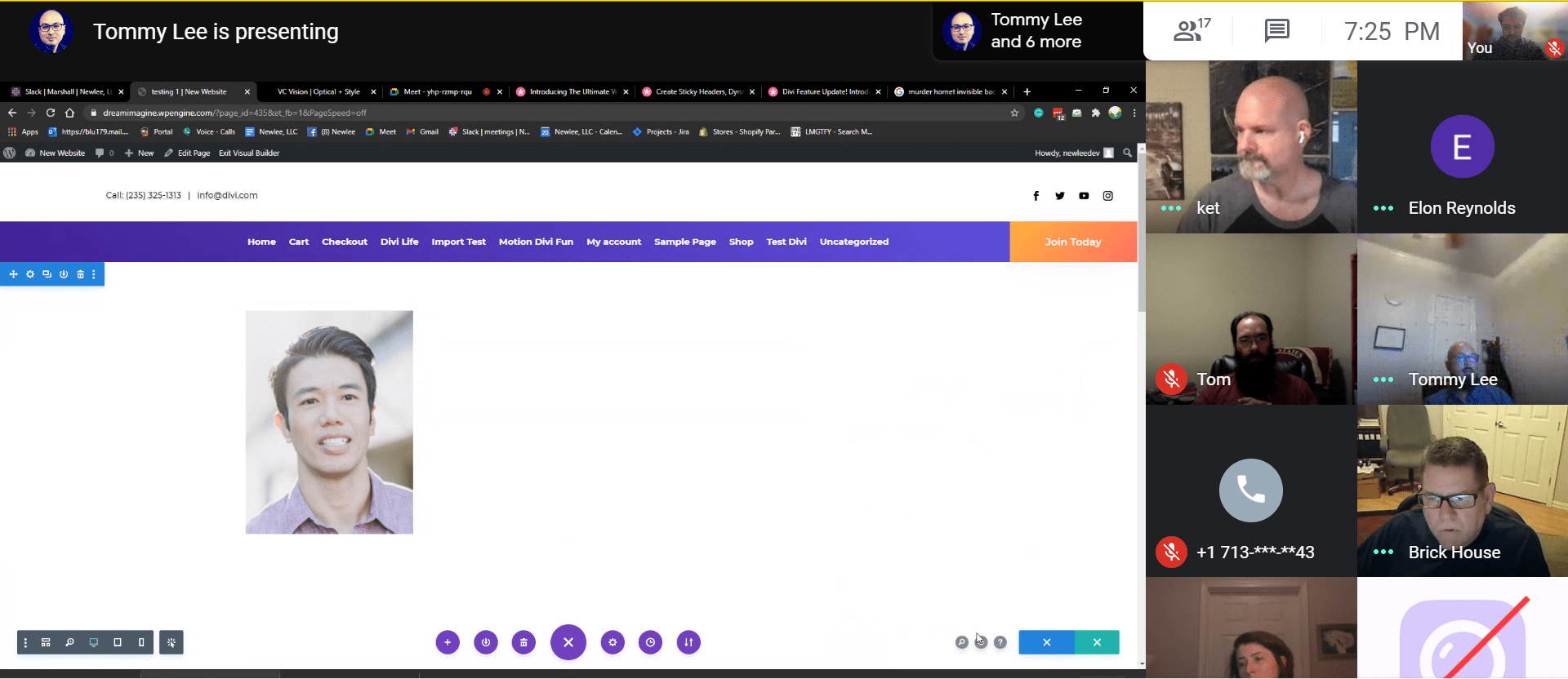The image depicts a multi-paneled online meeting or presentation interface with an array of participant thumbnails arranged systematically. Here’s a breakdown of the detailed observations:

- **Top Right Corner**: Above the top two participant images is a white bar displaying an icon of a person with the number "17" beside it, a chat icon, and the time "7:25 p.m."
  
- **Top Row**: 
  - **First Thumbnail** (left): A bald man with a goatee looking to the left.
  - **Second Thumbnail** (right): A blank screen with a purple circle featuring a white "Y." Text underneath reads "Alan Reynolds."

- **Second Row**:
  - **First Thumbnail** (left): A man with a beard and hair, sitting in a chair.
  - **Second Thumbnail** (right): Another man sitting in a chair against a white wall.

- **Third Row**:
  - **First Thumbnail** (left): A blank background (black) with a gray circle featuring a white phone icon.

- **Fourth Row**:
  - **First Thumbnail** (left): An older man with glasses and short hair in front of a white door.
  - **Second Thumbnail** (right): Images cut off halfway down.

- **Top Left Area**: 
  - A black-bordered icon of a bald man with glasses. To its right, the text reads "Tommy Lee is presenting."
  - Another instance of a similar profile picture, with text to the right stating "Tommy Lee" and "6 more."

- **Top Left Area Below**:
  - A series of drop-down tabs. The second one is highlighted in gray, while the rest are in black.
  - Directly below, a gray search bar spans across the image.
  - Below the search bar, a series of clickable links extend about two-thirds across the image.

- **Bottom Right**:
  - A white border containing a phone number, an email address, and social media icons for Facebook, Twitter, YouTube, and Instagram.

- **Bottom Section**:
  - A purple bar with white text near the left: "Home," "Car," "Checkout," "DVI," "Life," "Import," "Test," "Motion," "Divi Fund," "My Account," "Sample Page," "Shop," "Test," "Divi," and "Categories."
  - A green tab with white text reading "Join Today."
  - A picture of a man with short brown hair in the center. 
  - Lower section includes gray bars in the bottom corner, purple in the center, and both blue and green bars on the right side.

The detailed caption captures the essence of the image, providing insight into each segment, making the layout and elements vividly clear.